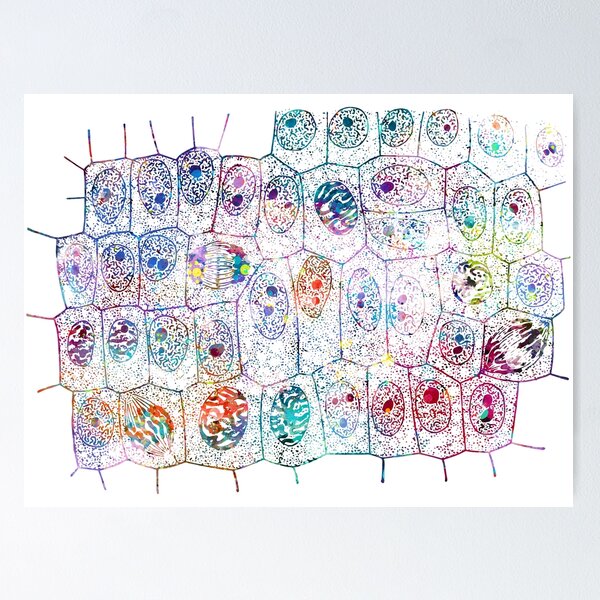This image is an intricate and abstract painting depicting a series of interconnected multi-colored cells, each reminiscent of a honeycomb pattern. Set against a gray background, the artwork features various cells placed on a white paper. The cells are portrayed as irregular, often egg-shaped boxes filled with an array of vibrant colors such as purple, blue, red, and yellow. Within each box, there is a central colored oval, often containing black dots that give the appearance of nuclei or eyes, lending some circles a face-like look. These central forms are surrounded by lines extending from the edges of the boxes, enhancing the interconnected nature of the design. The cells within the image seem to represent different stages of mitosis, with some showcasing condensed chromatin or nuclei in the process of division. Certain cells appear faded but maintain a multi-colored spectrum overall, contributing to a rainbow gradient aesthetic. This captivating blend of science and art conveys the dynamic beauty of cellular division, featuring detailed stages of mitosis in a highly stylized format.